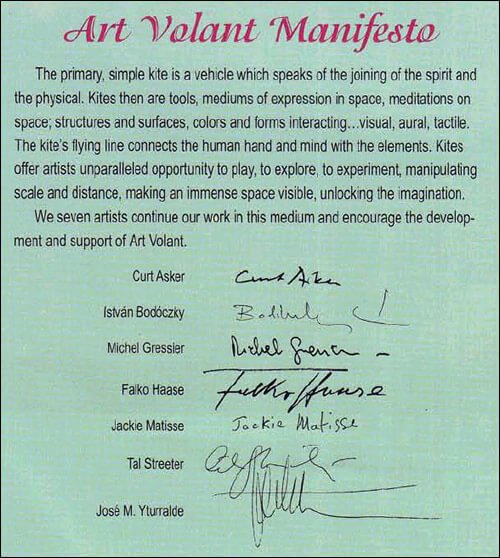The image displays a green piece of paper with a woven texture, titled "Art Volant Manifesto" at the top in a vibrant maroon-pink font. The text below is a detailed paragraph written in black, stating, "The primary simple kite is a vehicle which speaks of the joining of the spirit and the physical. Kites are tools, mediums of expression in space, meditations on space, structures and surfaces, colors and forms interacting, visual, aural, tactile. The kite's flying line connects the human hand and mind with the elements. Kites offer artists an unparalleled opportunity to play, to explore, to experiment, manipulating scale and distance, making immense space visible. Unlocking imagination, we seven artists continue our work in this medium and encourage the development and support of Art Volant." At the bottom of the document are the names and signatures of seven artists: Kurt Asker, Ysvan Badowski, Michael Gressier, Falco Haas, Jackie Matisse, Tal Streeter, and Jose M. Uralde.